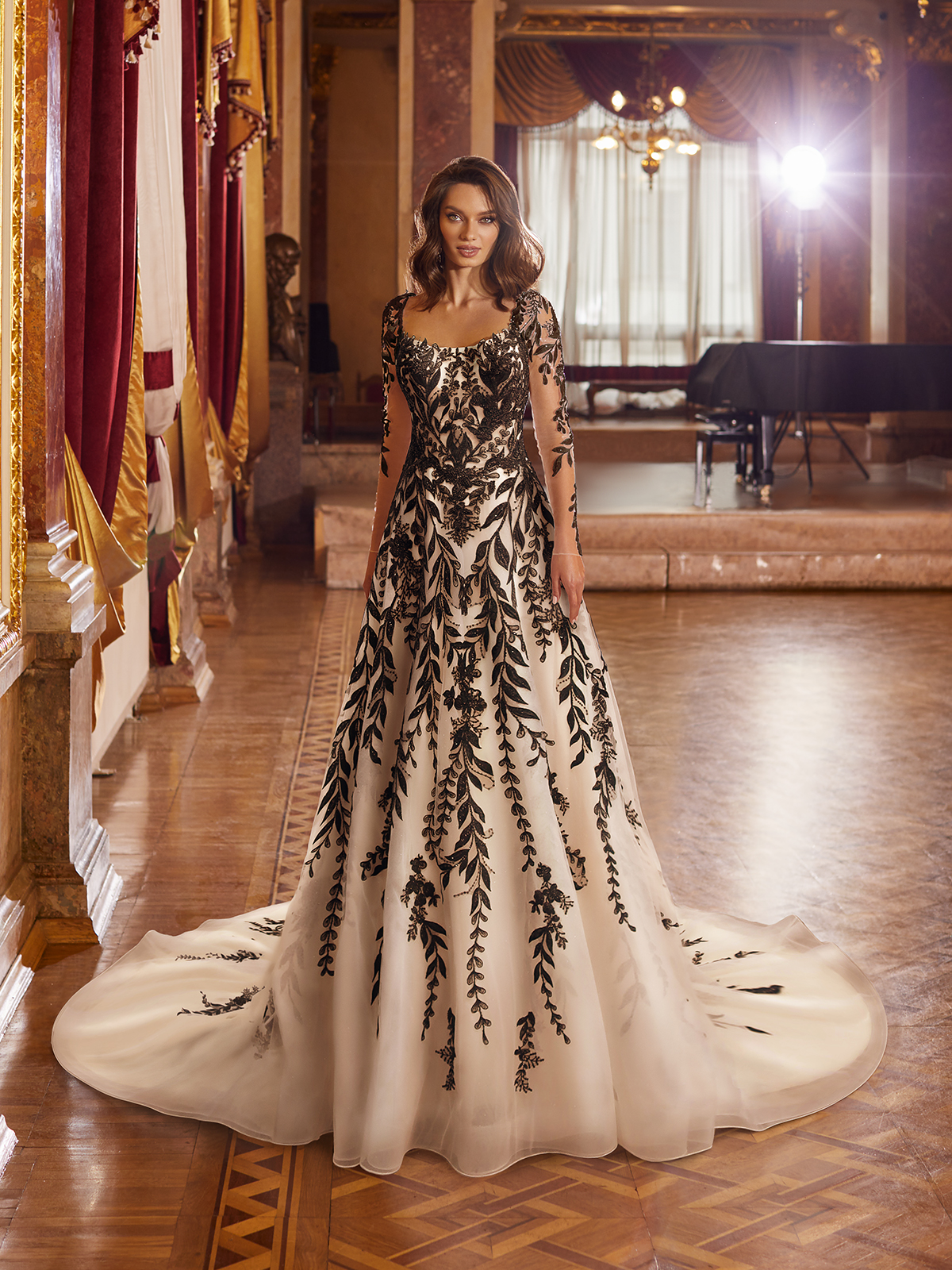In this detailed photo taken indoors, a large and opulent ballroom, reminiscent of a palace or a grand mansion, sets the scene with its luxurious and expensive decor. Dominating the center of the image, a woman with shoulder-length brown hair stands confidently on a wooden parquet floor. She has an olive skin tone and ethnic features, exuding elegance in a magnificent black and white ball gown. The dress, featuring a fitted bodice with an open chest area and partially transparent sleeves adorned with black floral leaves, transitions into a wide, circular train of white fabric intricately detailed with black vine patterns that thin out towards the hem. Behind her, a prominent wooden stage supports a black grand piano with a closed lid, situated beneath a spotlight. Large windows framed by dramatic deep red velvet curtains, lined with gold and complemented by white sheer curtains, further enhance the grandeur. The ornate carvings on the walls, alongside more red velvet curtains, complete the lavish environment that envelops the poised model.